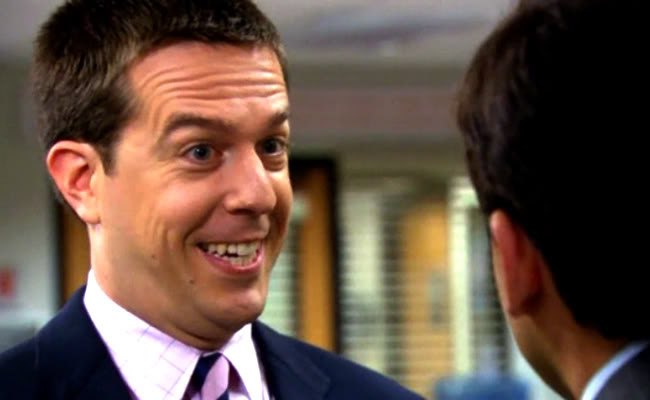The image appears to be a clip from a television show featuring two middle-aged men in an office setting. The man on the left, who has short black hair and is smiling with a forced expression, is dressed in a blue dress shirt over a light pink collared shirt, accessorized with a pink and black striped tie. His upper body is cropped out past the shoulders. On the right side of the image, partially visible, is another man with short black hair, slightly smaller in stature, wearing a black shirt with a white collar. The background is blurred, revealing an office area with large windows covered by white blinds and a hallway beyond.